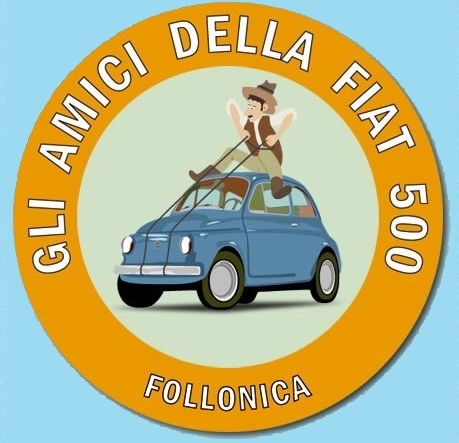The image features a round badge or decal with a light blue background and a prominent yellow outline. Inside the yellow circle, the words "Gli Amici Della Fiat 500" are inscribed around the top half, while "Follonica" is written at the bottom. At the center of the badge, a cartoon illustration depicts a man wearing brown and grey clothes, a vest, boots, and a hat. The man is seated on top of a small blue Fiat 500, using two reins attached to the front grille as if riding a horse. The overall design suggests a playful and whimsical advertisement or emblem for a group or community associated with Fiat 500 enthusiasts.